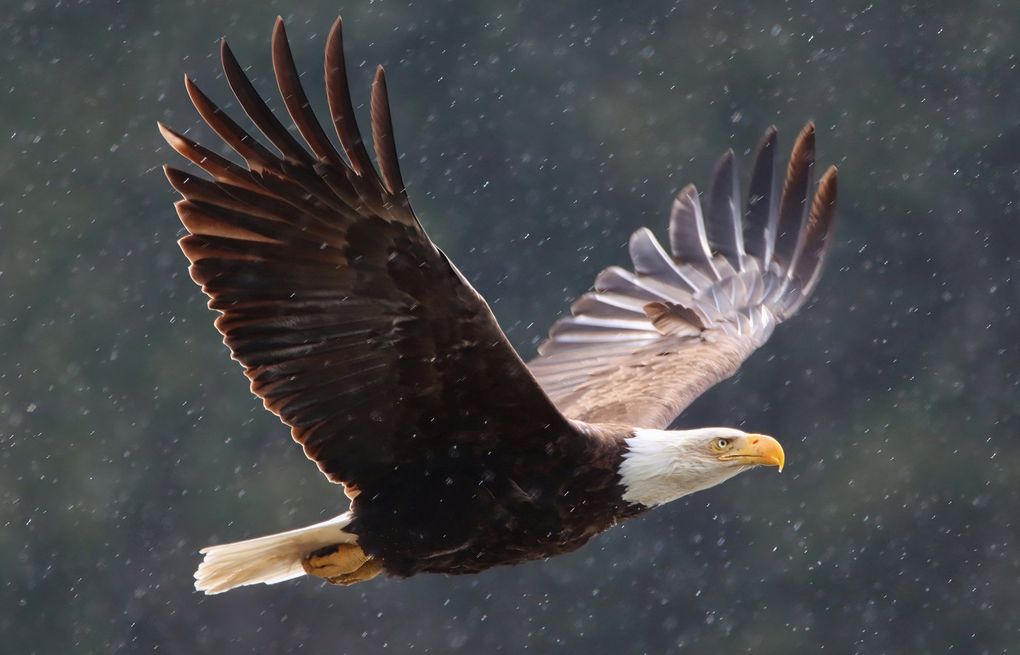A mesmerizing photograph captures a majestic bald eagle soaring through a snowstorm with its wings fully outstretched, dominating the image from front to back. The eagle's fierce, determined gaze is directed towards the right, accentuated by its striking yellow eye and sharp, yellow-orange beak. The pure white feathers on its head contrast vividly with its dark brown body feathers, which take on an almost grayish hue from a distance. Its powerful talons, a lighter orange, are tucked under its body for streamlined flight. Each individual feather of its expansive wingspan is clearly visible, emphasizing its powerful presence. The background, a blurred mix of dark gray and green, is dotted with falling snowflakes, adding to the dramatic and wild beauty of the scene. The eagle, smaller than a full-fledged adult, exudes an air of majestic determination and hunting prowess.